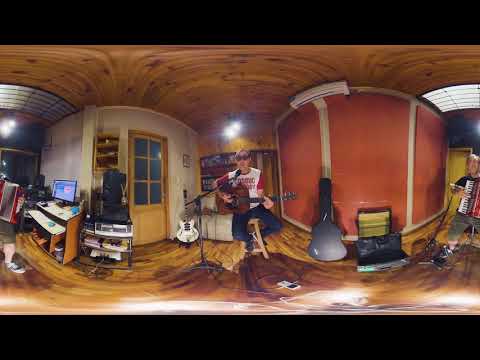In this intriguingly distorted photographic image, likely taken with a wide-angle lens, three men are seen performing indoors, possibly in a recording studio or someone's basement repurposed for musical practice. The lens causes everything to appear curved and slightly surreal. Center stage is a white man wearing a red and white short-sleeve t-shirt, blue jeans, and black glasses. He is seated on a wooden barstool, strumming an acoustic guitar and singing into a microphone mounted on a stand. To his right, a white man is playing an accordion while dressed in a dark shirt and green pants. Flanking the central figure on the left side, only the legs of another man, clad in green shorts and sneakers, are visible, also playing a red accordion.

The backdrop reveals a myriad of musical equipment: between the central and right figures, an acoustic guitar leans against a red wall with a black case beside it. To the left of the central performer, an electric guitar stands on a mount next to a shelving unit filled with various equipment, books, and a computer desk setup. The room features a brown ceiling and matching floor, and a door with six glass panels stands to the left of the main performer. Despite some text on the center man's shirt, it remains unreadable. This colorful and cluttered photo captures the essence of a lively, makeshift studio, where music and creativity are in full flow amidst a visually intriguing space shaped by the lens's distortion.